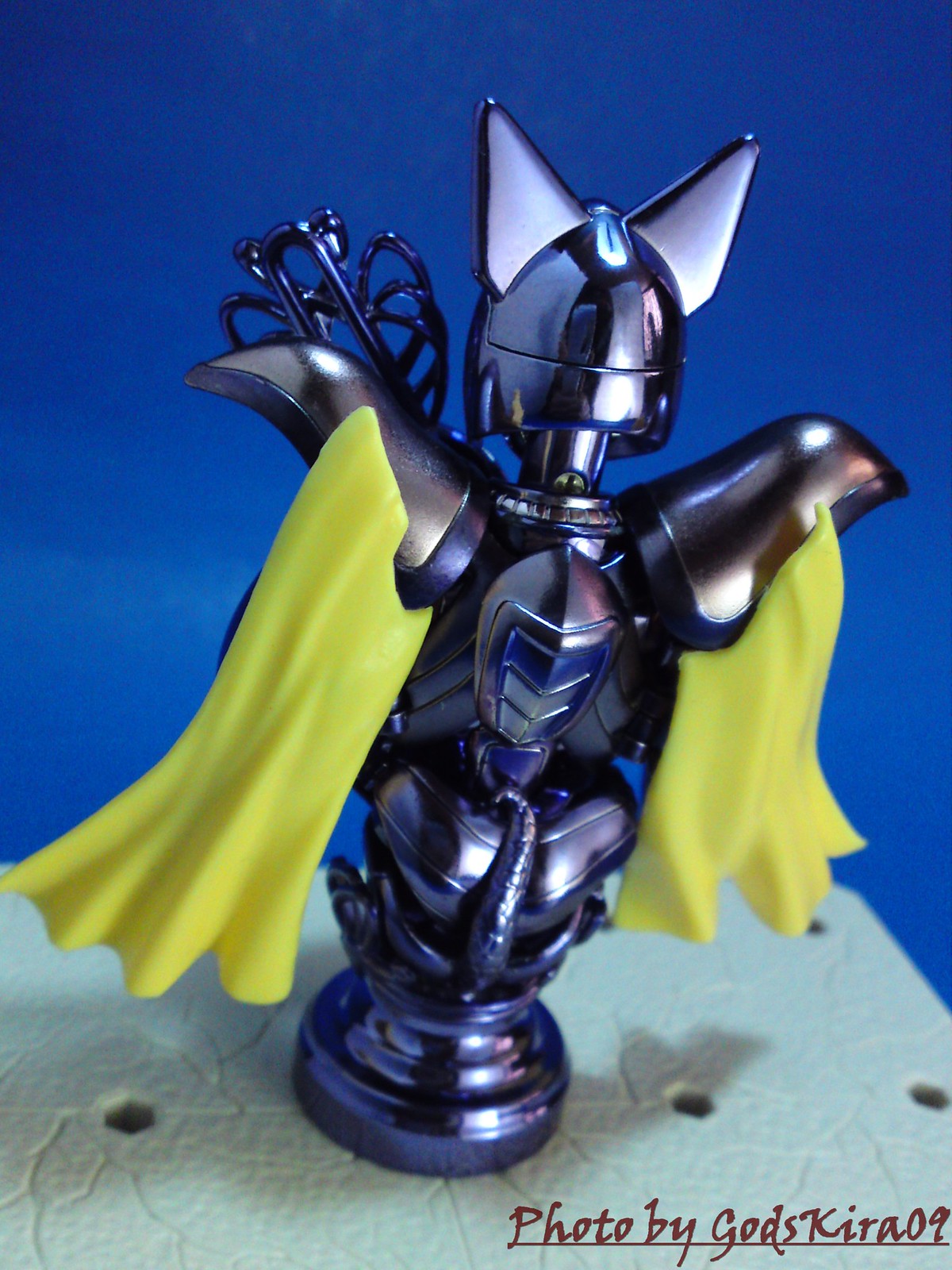In this vibrant photograph by Godskira09, a striking metallic sculpture of a superhero cat stands prominently against a rich, dark blue background. The cat figure, crafted from gleaming metal in shades of shiny gray and blue, features distinctive cat ears atop a helmet-like head that is split in the center. With arms raised and embellished with yellow flaps that mimic a cape or flowing material, the feline superhero exudes a sense of motion and action. The body includes intricate details like a scaly tail that curves upward, suggesting the back view of the figure.

The sculpture is mounted on a white ceramic or plastic base, which has a granulated texture and several small holes that may hold action figures securely. Four screw holes are visible, indicating how the sculpture is affixed to the round pedestal. The pedestal, detailed with cracks and a stone-like appearance, serves as a stable platform for the figurine. At the bottom of the image, in the lower right-hand corner, the credit "photo by Godskira09" is displayed in a brown font, neatly underlined, emphasizing the artist's contribution. The overall dimensions of the photo are approximately six inches high and four inches wide, perfectly capturing the intricate details and the dynamic presence of this superhero cat sculpture.